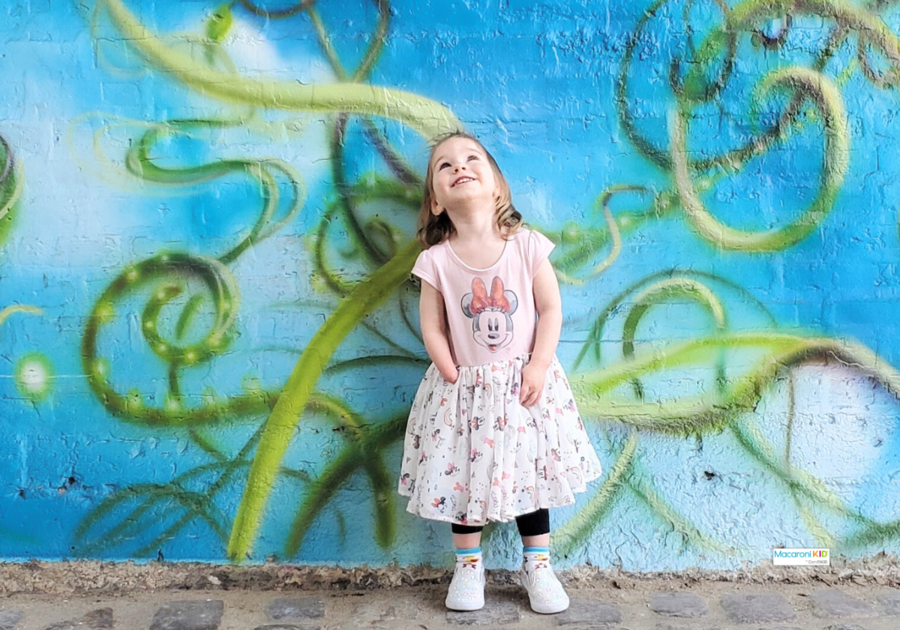The photograph, taken outdoors during the daytime, captures a heartwarming moment of a young girl, approximately two to three years old, with light brown shoulder-length curly hair. The girl is of lighter complexion and is smiling brightly, gazing upward with her head tilted back, revealing the underside of her chin and showing her teeth.

She is dressed in a charming pink dress featuring a classic-style Minnie Mouse illustration on the front, with Minnie sporting a red bow. The dress has short sleeves and transitions into a nearly-white pink skirt adorned with multiple Minnie Mouse heads. She is also wearing black leggings underneath her dress, white shoes, and white socks with a blue rim at the top and possibly yellow flowers printed on them.

The background of the image is a stone brick wall that has been painted blue with whimsical white clouds and green vines spiraling up the side. The vines, intertwined with lights, add a playful touch to the scene, which appears to feature graffiti art. At the bottom right corner of the image, there’s a logo that reads "Macaroni Kid" in colorful blue, orange, purple, and green lettering.

The setting of the photograph is well-lit and clear, emphasizing the vibrant and joyous atmosphere surrounding the little girl as she enjoys this moment outdoors.